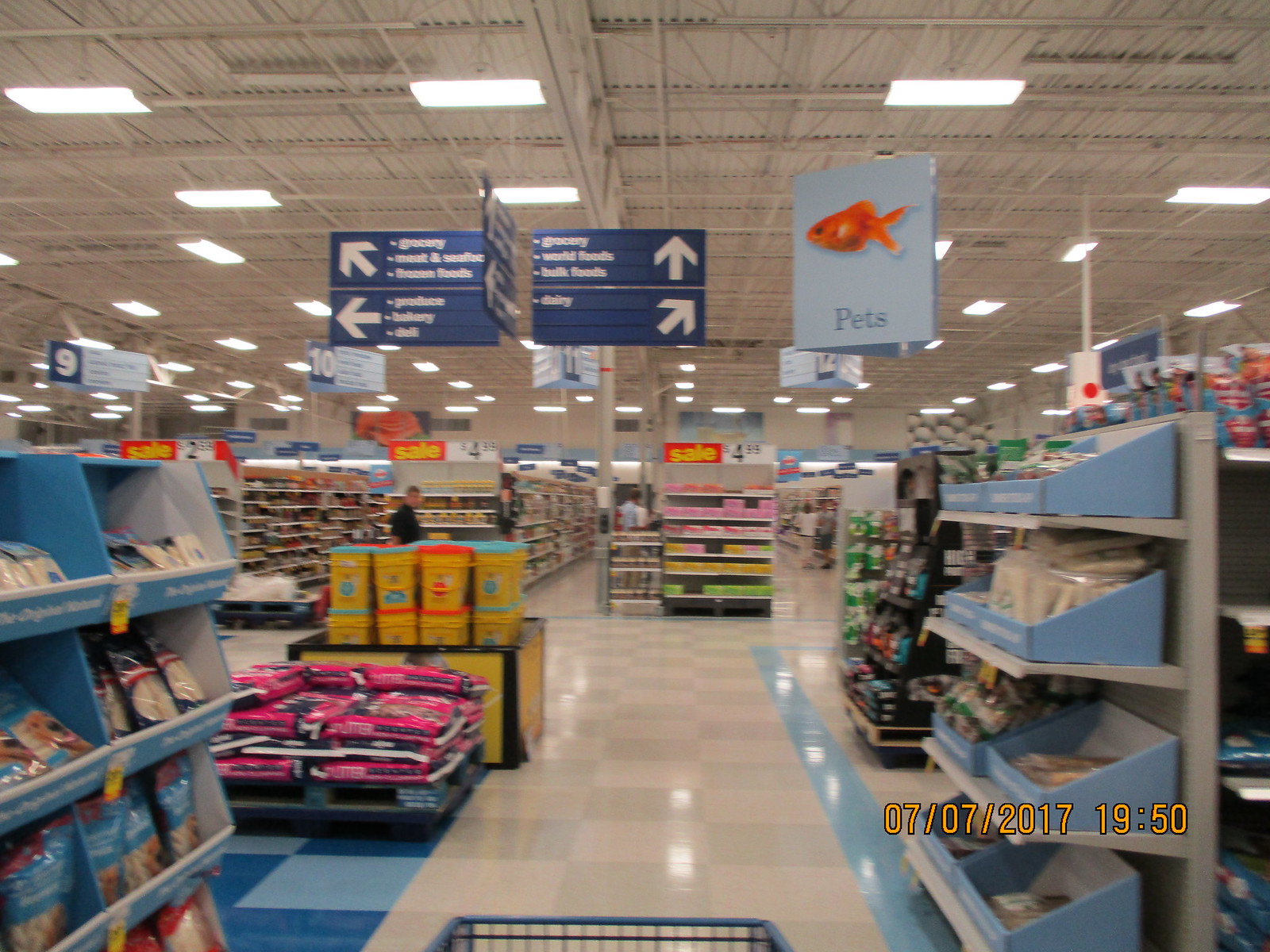This image captures the point of view of someone pushing a blue shopping cart, dated July 7, 2017, at 7:50 PM, likely in a department store similar to Walmart. The perspective shows the shopper navigating through wide, tiled aisles. Blue pallets display pink bags of dog food to the mid-left, with yellow gallon-sized containers of Tidy Cat litter further down the aisle. Above, a network of metal beams supports rectangular white lights, illuminating signs overhead directing customers towards various sections like groceries, bakery, deli, produce, and dairy. Prominently, a large light-blue, triangular-shaped sign marked “Pets” with an image of a goldfish designates the pet supplies area, grounding the scene in a high-traffic, organized retail environment.